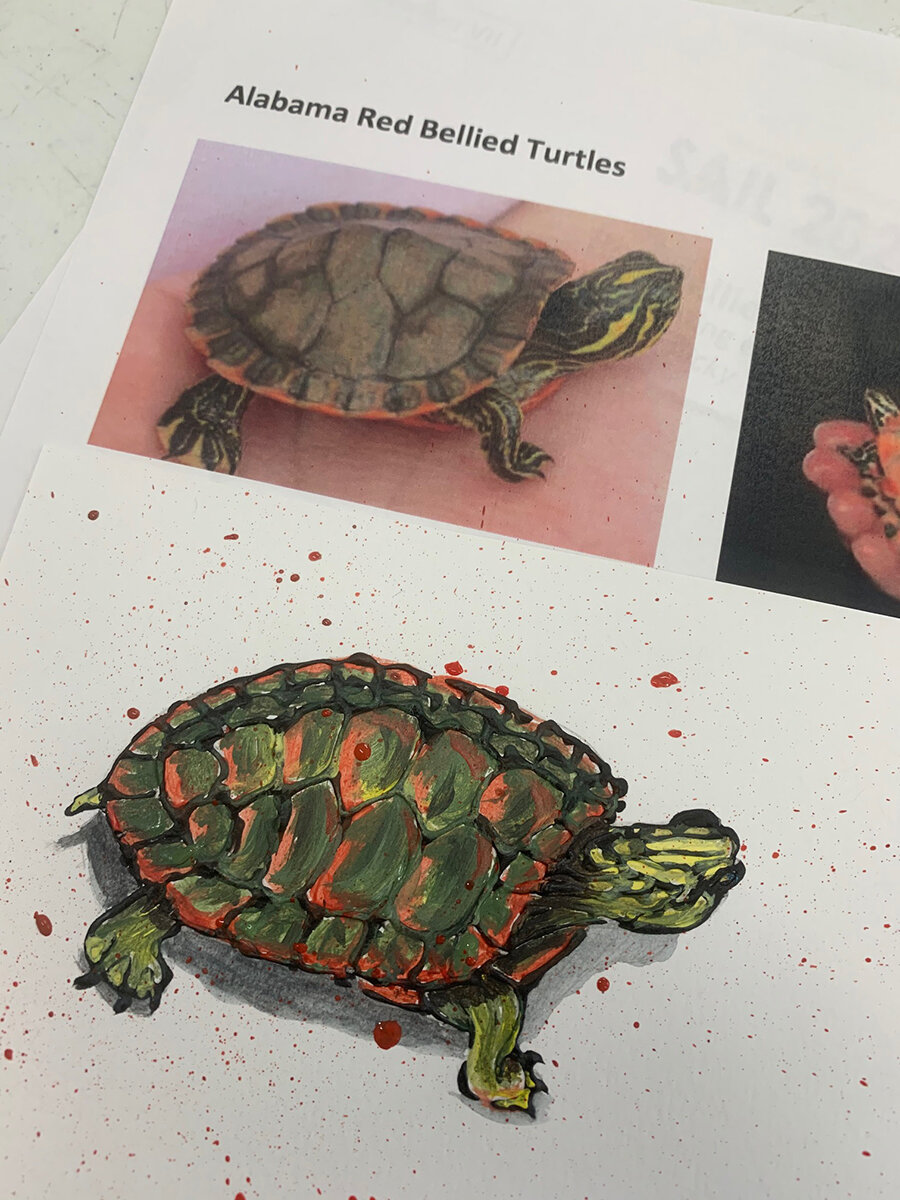In this image, sourced from a textbook page, the focus is on the Alabama red-bellied turtle. The page contains three visuals: at the top left, there's an actual photograph of the turtle, accompanied by the caption "Alabama red-bellied turtles." Adjacent to this, partially off-screen, is a second image depicting the turtle being held in a human hand, giving a sense of its small size. The turtle's body features a mix of green with slight touches of red and orange, particularly visible on its shell. Below these, on the white paper canvas, an artist has recreated the turtle from the photograph, meticulously matching the colors and details. The painting includes a speckled background with rust-red paint specks, some of which have found their way onto the turtle depiction itself. The artist has paid careful attention to individual elements like the black and yellow patterns on the turtle's head and legs, capturing the essence of the Alabama red-bellied turtle as detailed in the textbook.